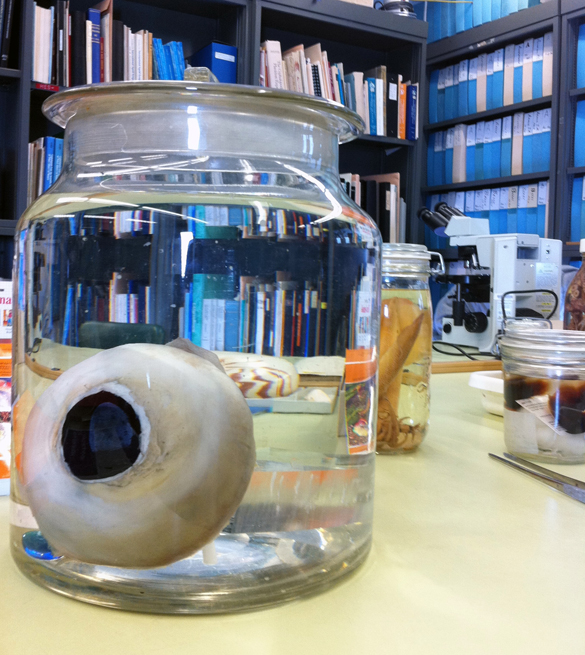In this image, several glass jars filled with various objects are prominently displayed, with one large, clear jar in the center housing an off-white, dirty-looking object resembling an eyeball. This distinct object features a black center encircled by a brighter white ring. The jar is filled with liquid, allowing visibility through to the background. Behind it, bookshelves lined with colorful binders and books, primarily blue, black, and white, can be seen, indicating a library or research setting.

Additional smaller jars flank the central one: the middle-sized jar contains an orange object, while the smallest jar has a dark brown substance suspended in it. Also present on the right side of the image is a microscope, further suggesting a scientific environment. The scene appears to be set on a desk in what could be an office or laboratory, emphasizing a focus on biological or anatomical research.